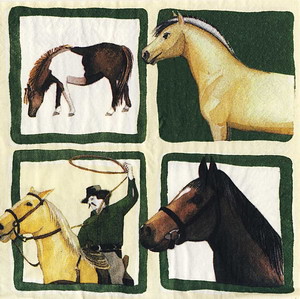This detailed illustration features four distinct horse scenes arranged in a square grid with green backgrounds, resembling a window with four equal panes. The upper left pane depicts a brown and white horse, identified by its brown head, neck, and back, grazing peacefully. Adjacent to it in the upper right pane, a golden yellow horse with a white mane is positioned as if its head is emerging from the edge of the frame. The lower left pane shows a dynamic scene of a cowboy in a long-sleeved green shirt and black hat, brandishing a lasso while riding another yellow horse. Finally, in the lower right pane, a dark brown horse is seen with its neck and head sticking out, distinguished by a white spot between its eyes.